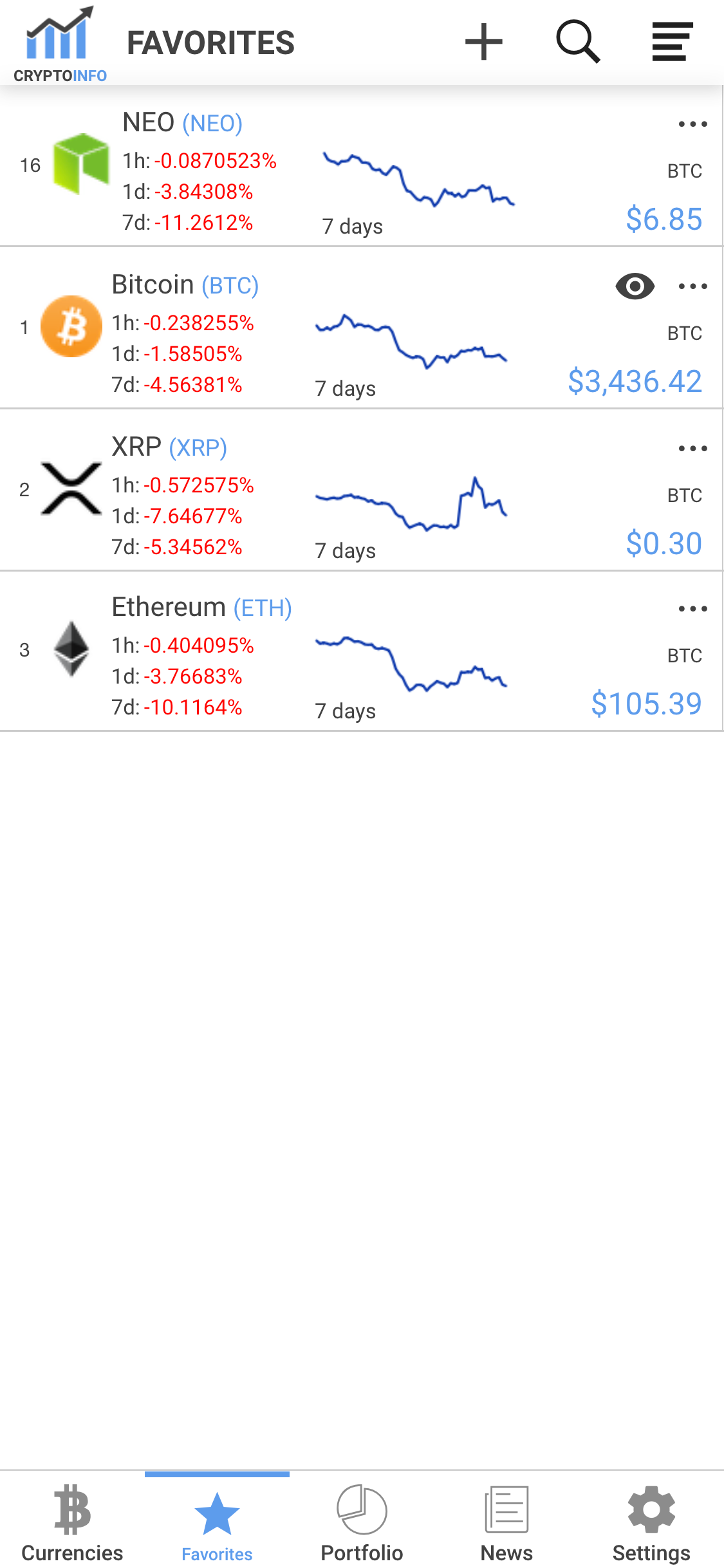This screenshot captures a user interface from a cryptocurrency tracking app or website. At the top of the interface, there is a white horizontal bar. In the left corner of this bar, the text "Crypto Info" is displayed next to a blue bar graph icon with a gray arrow overlay. To the right, it reads "Favorites." Adjacent are icons for adding items (a plus sign), searching (a magnifying glass), and accessing a menu (four horizontal lines forming a drop-down menu).

Beneath this section lies the main display area, featuring four different cryptocurrency graphs with their respective performance indicators. The first cryptocurrency, NEO, is represented by an open green cube logo. The graph for NEO generally trends downward and includes valuation data over one hour, one day, and seven days, with a current value of 6.85.

Next is Bitcoin, which shows a graph that remains relatively stable before dipping and then experiencing a slight recovery. Following Bitcoin is XRP, illustrated with a graph that declines initially, flattens out, surges significantly, and then drops slightly again. Finally, there's Ethereum, whose graph starts high, trends downward, shows a modest recovery, and then ascends once more.

Each cryptocurrency is accompanied by percentage change data for one hour, one day, and seven days, all presented in a highly organized and reader-friendly format, making it easy to track and compare their performances at a glance.